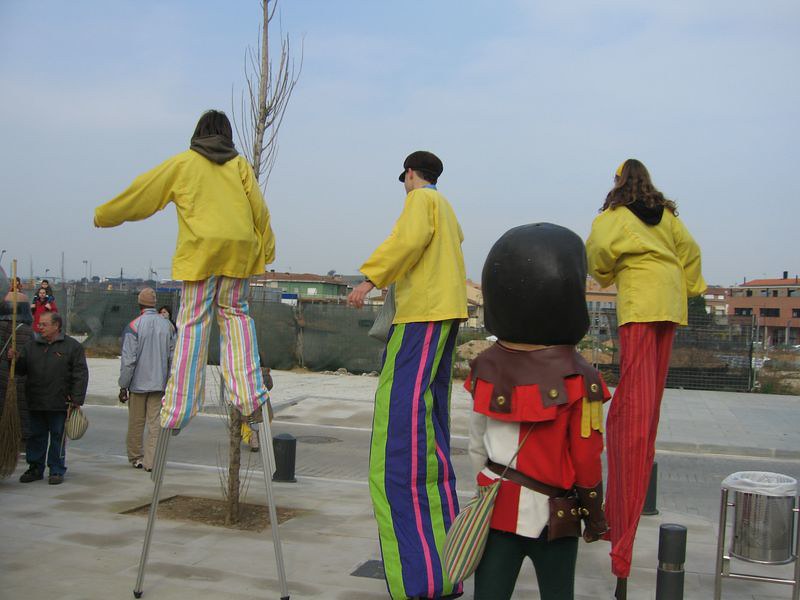In this outdoor photo, taken during a cold time of the year as indicated by everyone wearing heavy jackets, there are three individuals walking on stilts and one person in a costume, all set against a backdrop of tall buildings and a white sky. All three stilt-walkers are dressed in distinctive yellow slicker rain jackets.

On the center left, a person wearing vertically striped pink and light blue pants, which reveal the stilts they are standing on, has their hands tucked inside the jacket, and their black hood sticks out the back. The center of the image features a man with a light complexion and long vertically striped pants in light green, purple, and pink, which conceal his stilts. He wears a black-billed cap and is also wearing the yellow slicker. To the right, another stilt person is seen with reddish pants that have light white stripes, their stilts just peeking out from under the pants. This person has long brownish-black hair and a hint of a yellow scarf at the front.

Amidst these towering figures stands a shorter individual dressed like a medieval character, complete with an oversized helmet resembling a Prince Valiant haircut. This figure, clad in a red and white checkered shirt, a black belt, and a brown pouch on the right hip with a small bag slung over their shoulder, adds an element of theatricality to the scene.

They all are walking on concrete where a few black devices or fixtures protrude from the ground. A man in a grey jacket holding a giant broom can be seen nearby, enhancing the bustling ambiance of this whimsical moment.